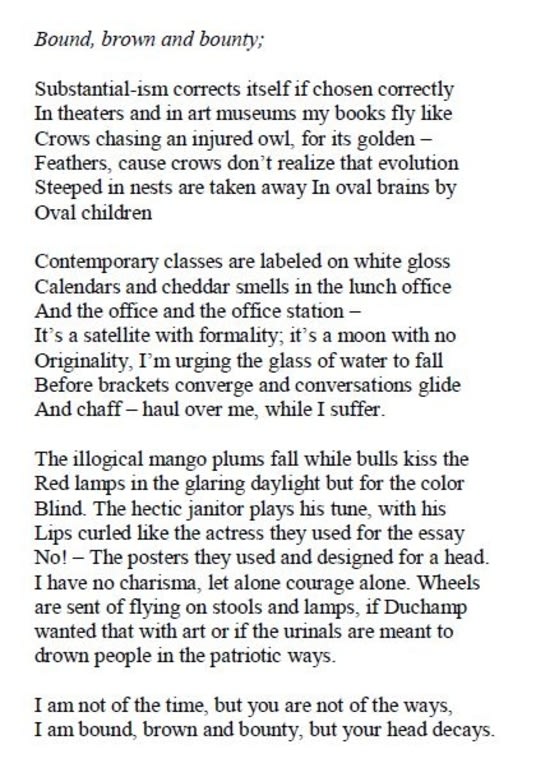The image showcases a scanned piece of text, likely a poem titled *"Bound, Brown, and Bounty."* The poem opens with the line, "Substantialism corrects itself if chosen correctly," suggesting an exploration of philosophical themes. It describes scenes both in theaters and art museums, where the author’s books are likened to crows chasing an injured owl for its golden feathers—a metaphor for relentless pursuit. The text underlines the irony that crows fail to recognize how evolution, deeply embedded in nests, is co-opted by the younger generation's undeveloped minds.

Contemporary classes are methodically scheduled on white-gloss calendars, contrasting sharply with the trivial cheddar smells in the lunch and office areas, highlighting mundane daily life. The narrative continues, portraying a formal yet unoriginal atmosphere described as "a satellite with formality and a moon with no originality." The poet urges for symbolic action, like “the glass of water to fall before brackets converge,” signifying an impending collapse of order.

As the poem progresses, images of "ecological mango plums" and "bulls kissing red lamps in glaring daylight" create a surreal landscape, emphasizing the chaotic and almost apocalyptic themes under a facade of normalcy, reflective of the colorblind's perspective. The hectic janitor, an Everyman figure, plays a melancholy tune with lips curled reminiscent of an actress used in an essay or a poster, as the poet reflects on their own lack of charisma and courage.

Further, the poem captures the descent into absurdity with "wheels sent off flying from stools and lamps" and questions the artistic merit and purpose of objects like urinals in a patriotic context. Finally, the poet concludes by confronting personal and temporal disconnection, stating, "I am not of the time, but you are not of the ways. I am bound, brown, and bounty, but your head decays."